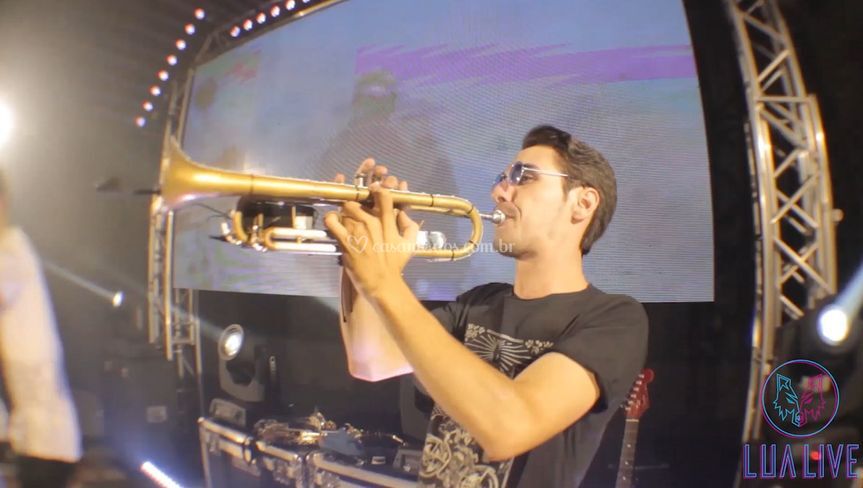In the foreground of this fish-eye angle image, a man in his 30s, with short brown hair and eyeglasses, is centered, passionately playing a gold and silver trumpet. His short-sleeve black shirt features a graphic partially obscured by his bent arms. The trumpet's tip is pressed against his lips, and his fingers are actively pressing the valves, indicating he's in mid-performance. The background reveals a blurred large projector screen displaying indistinct images, framed by solid black corners. This setup suggests he is on a stage. Visible lighting and steel girders above, alongside illuminated spotlights on a table below the screen, imply an ongoing concert, potentially an outdoor music festival. Additional stage equipment and a guitar case with a brown end can be seen in the periphery. Prominently displayed in the lower right corner, a circular logo with a wolf face, outlined in blue and purple, encircles the text "LUA LIVE" in vibrant purple letters.